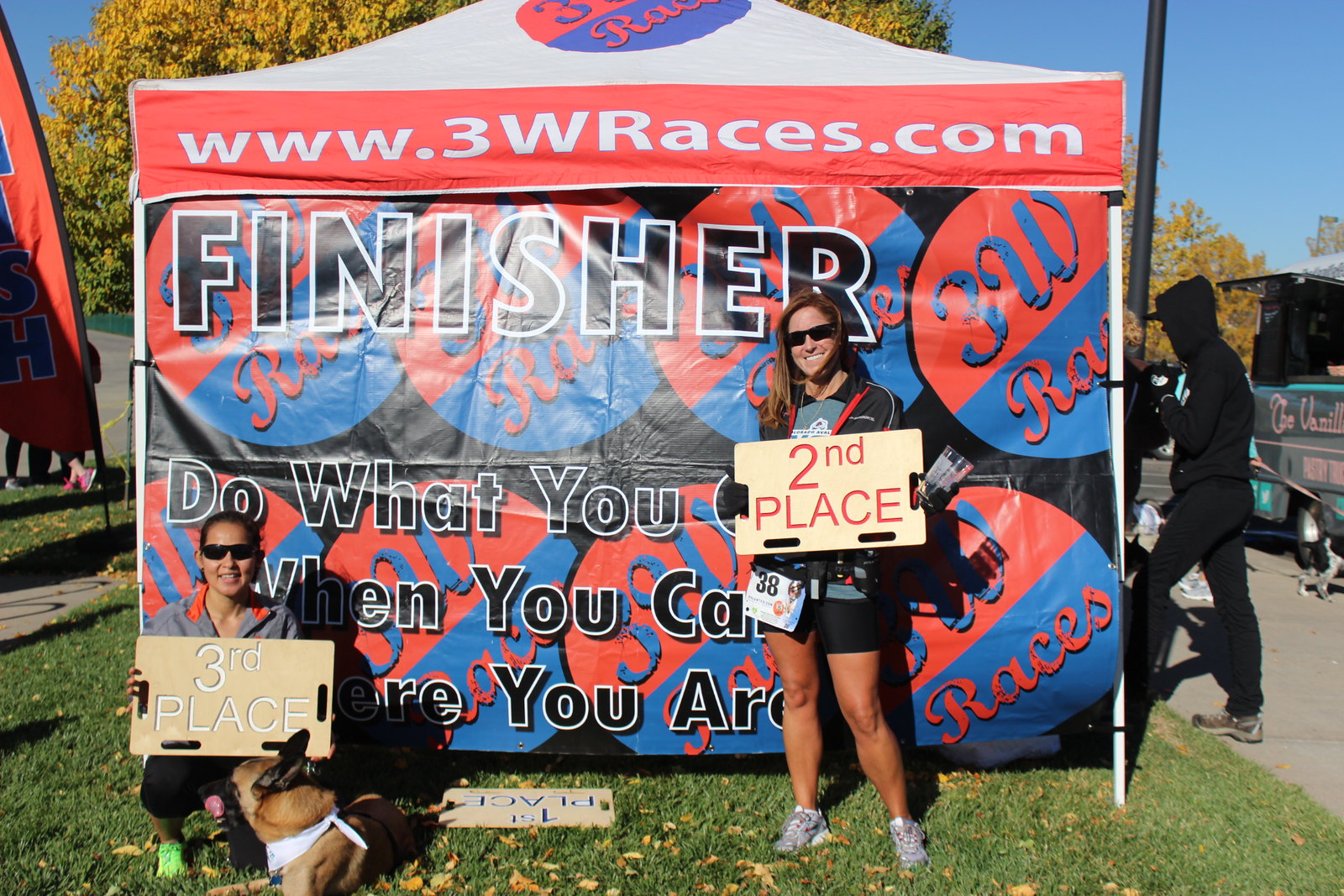In this vibrant outdoor scene set against a clear blue sky and the backdrop of colorful fall foliage, two young women, apparently having just finished a running race, are prominently featured. They stand in front of a tent emblazoned with "www.3wraces.com" in bold white letters on a red background. Stretching across the front of the tent is a large banner in red and blue that reads "3Wraces," with an inspiring message in black text overlaying it: "Finisher: Do what you can, when you can, where you are."

The runner on the left is squatting down, proudly displaying a white sign that proclaims her 3rd place finish. She wears sunglasses and her race tag number is visible. Beside her, lying on the grass, is a small dog attentively looking up at her. The runner on the right stands tall, also wearing sunglasses, and holds a wooden sign with red letters announcing her 2nd place victory. She is identified by a tag numbered 38. At their feet, a blue sign indicating the 1st place is laid on the ground, suggesting that the winner did not stay for the photo.

Adding to the scene, a person dressed in a black hoodie and black pants stands to the right of the tent, contributing to the bustling activity around this race event.